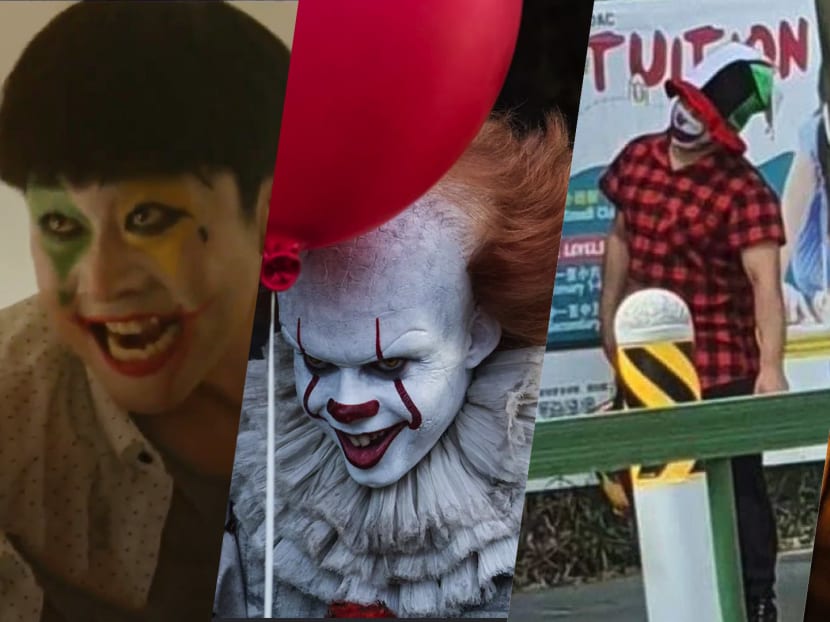The image depicts three human faces side-by-side, each adorned in distinct clown makeup, creating an eerie and unsettling theme. 

On the far left, a man with Oriental features sports clown-inspired makeup that includes red paint around his mouth, a green diamond surrounding one eye, and a yellow diamond around the other. His hair is styled in a short, bowl-like cut, and he wears an open white shirt with small polka dots over a gray t-shirt. His mouth is agape, giving him a menacing appearance, suggestive of an eccentric clown figure.

The middle figure is a more traditional, yet malevolent clown, with a fully white-painted face. His red lips and nose are accentuated with red paint that stretches above his eyes, which are further intensified by heavy mascara, giving him a sinister look. He has a broad, frilly white collar typical of clown attire, and his red hair flares out from a bald center, reminiscent of the classic "evil clown" or joker archetype.

On the far right stands a man in a red and black plaid shirt, complemented by a top hat that is black and green. His face is painted white, with red detailing around the lips and nose, resembling a grotesque smile. He's positioned in front of a truck and a green fence, possibly connected to a carnival setting, enhancing the sinister ambiance. His pose, along with the setting, gives off zombie-like, stumbling vibes, further contributing to the eerie, carnival atmosphere.